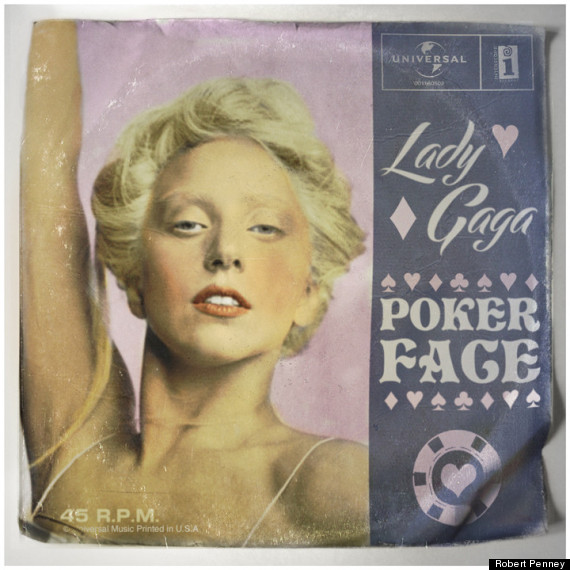This is a detailed depiction of a visually striking piece made to resemble a poster, album cover, or fabric tapestry segment. The image is square and appears slightly wrinkled, suggestive of a cloth material. The background is predominantly pink, giving the piece a retro and vibrant feel.

Featured prominently on the left side is Lady Gaga, styled with short, wavy blonde hair and bold red lipstick. Her pale skin contrasts sharply with the background, and she gazes directly at the viewer with squinting eyes, exuding confidence. Her pose is dynamic, with one hand raised. Only her upper body, from the neck up, is visible.

The right side of the image is adorned with text and motifs. At the top, "Universal Studios" is clearly visible, accompanied by a star and a diamond. Below, "Lady Gaga" and "Poker Face" are written, surrounded by light pink playing card suits, emphasizing the theme of the song. Additionally, there is a prominent pink poker chip toward the bottom right.

In the bottom left corner, the text reads "45 RPM," indicating the record speed commonly associated with vinyl records. Just beneath, it notes "Universal Music printed in the USA," which might hint at its distribution details. Overall, the image combines elements of music, artistry, and vivid color to create a captivating promotional piece for Lady Gaga's iconic track, "Poker Face."